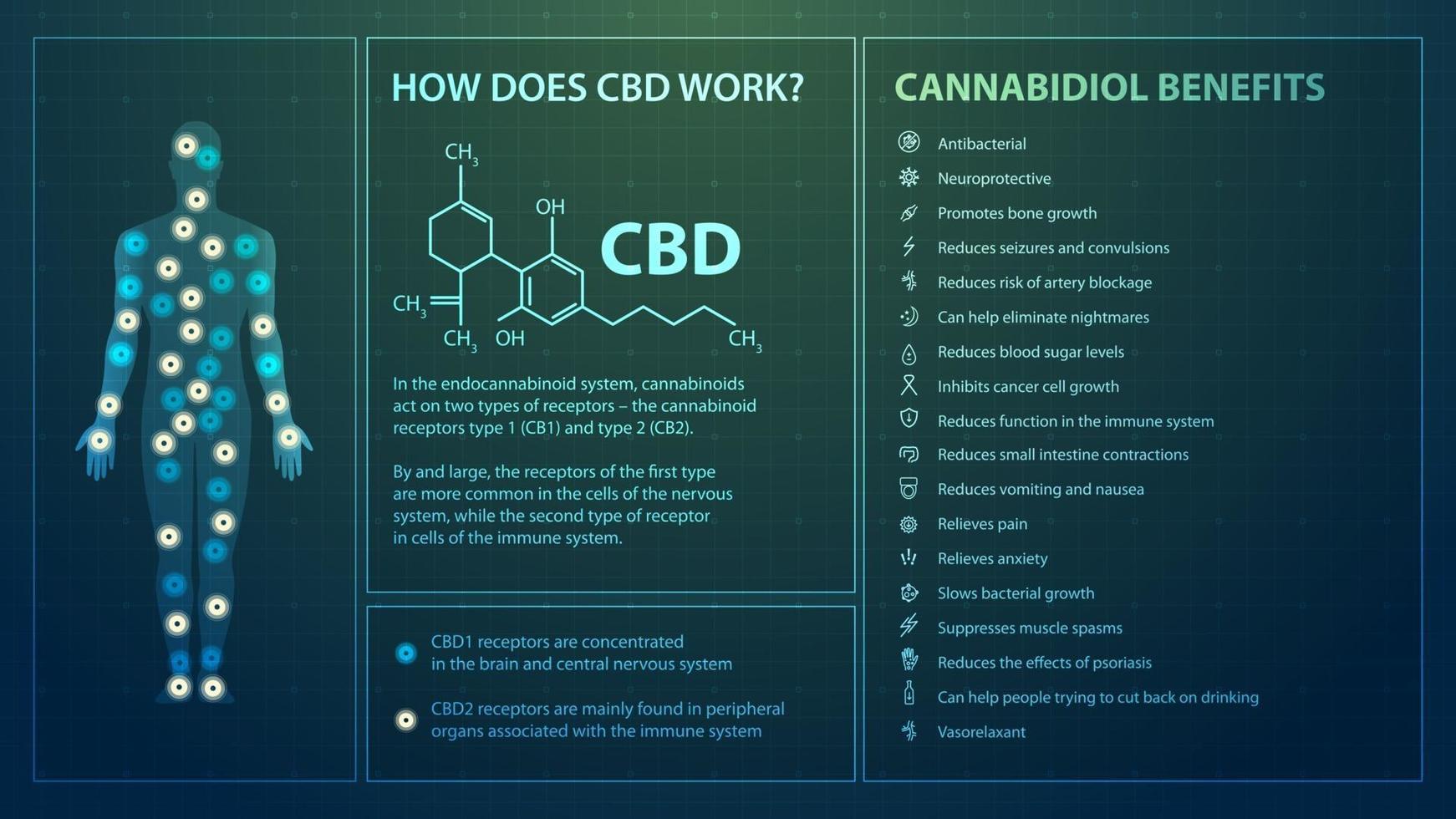This is an informational diagram explaining how CBD works, divided into three parts. On the left, a human silhouette highlights various points on the body with circular spots in blue and cream colors, representing CBD1 and CBD2 receptors, respectively. In the middle section, titled "How Does CBD Work," a chemical structure of CBD is depicted, along with an in-depth explanation of its interaction with the endocannabinoid system. It details that CBD1 receptors are primarily found in the brain and central nervous system, while CBD2 receptors are mostly located in peripheral organs linked to the immune system. The final section on the right lists the extensive benefits of cannabidiol, including antibacterial properties, neuroprotection, promotion of bone growth, reduction of seizures and convulsions, decreased risk of artery blockage, and numerous others, all accompanied by small illustrative icons.